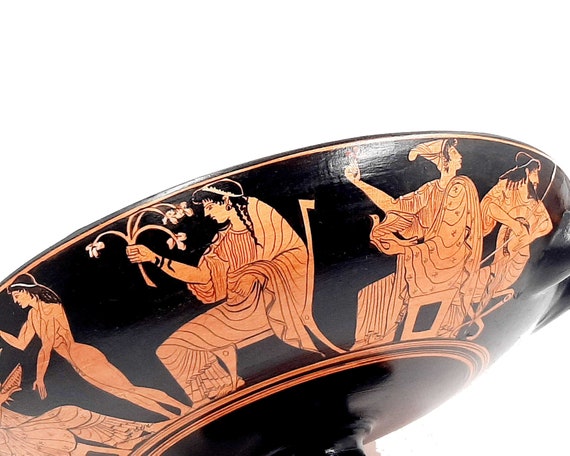The image showcases the underside and side of a black bowl, set against a completely white background. The bowl is slightly tilted, lower on the left side, and cropped on the left and right edges. The bowl features orange striping around the bottom edge. Along the side, there are intricately detailed, old-fashioned images depicting people in shades of orange and light orange, with black hair. One central figure, seated in a chair, is holding several drooping flowers. Behind him, two men look in the opposite direction. To the right of the seated man, another person stands. Additional figures include a naked man with outstretched arms and a cloaked individual holding a bird, changing into a serpent from the waist down. The scene is quite ornate and appears to be a classical or ancient depiction, adding to the bowl’s unique visual appeal.